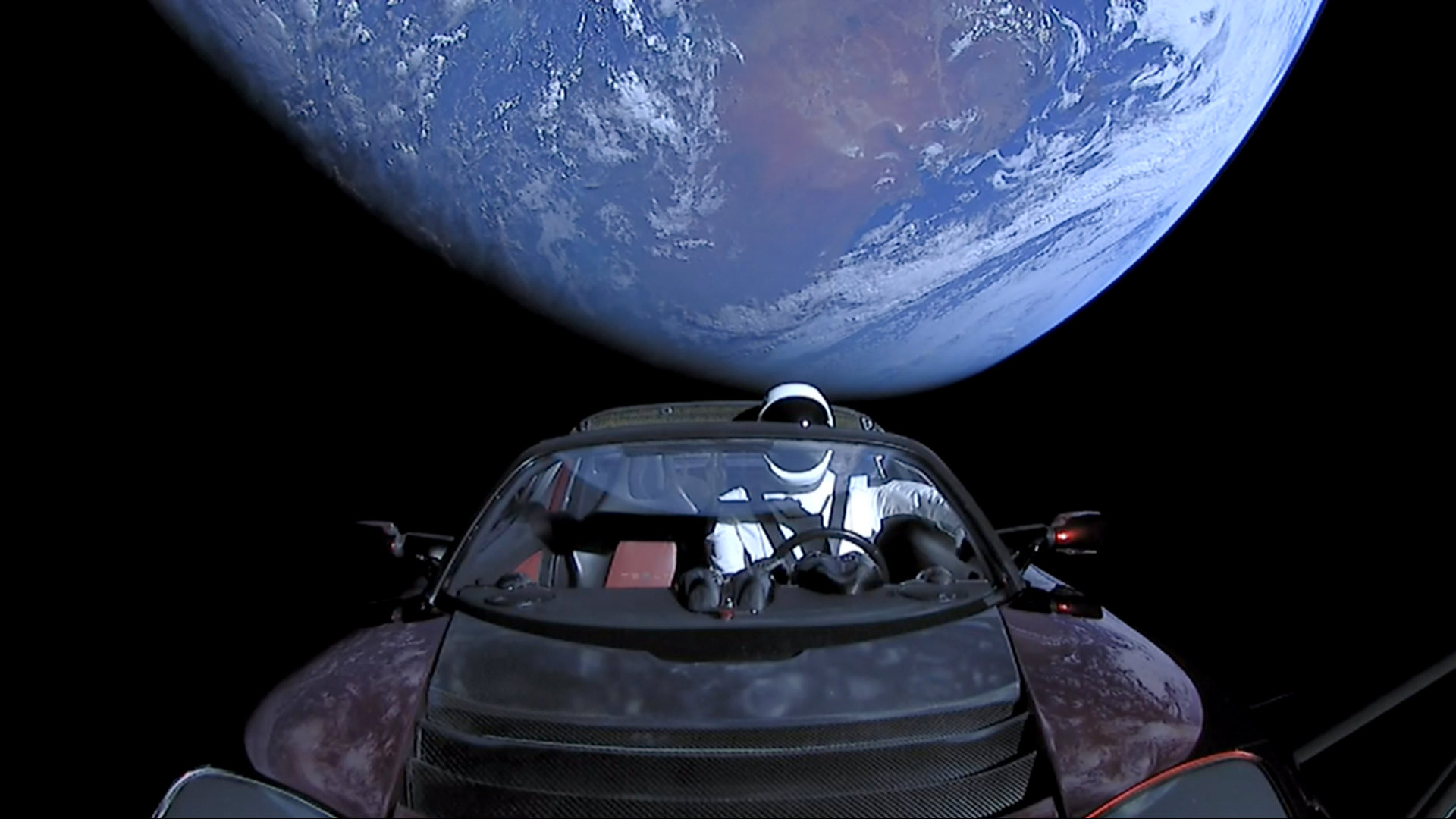This image showcases the famous Tesla car that Elon Musk launched into space, featuring a mannequin dressed like an astronaut, known as "Starman," positioned behind the wheel. The dark gray or black car, with lighting that gives it an almost purple hue in parts, is depicted floating above the Earth with its continents, clouds, and the vast expanse of space visible in the background. The car, which has an open roof, is meticulously detailed with elements like the steering wheel, side mirrors, and dashboard. Notably, the mannequin in a white astronaut suit has its arm hanging out of the window, giving a relaxed and casual impression as it floats in the cosmos. The realistic scene captures both the awe of space travel and the whimsical idea of a car cruising through the universe, blending elements that lead some to believe it could be digitally generated or photoshopped, though it is an actual photograph.